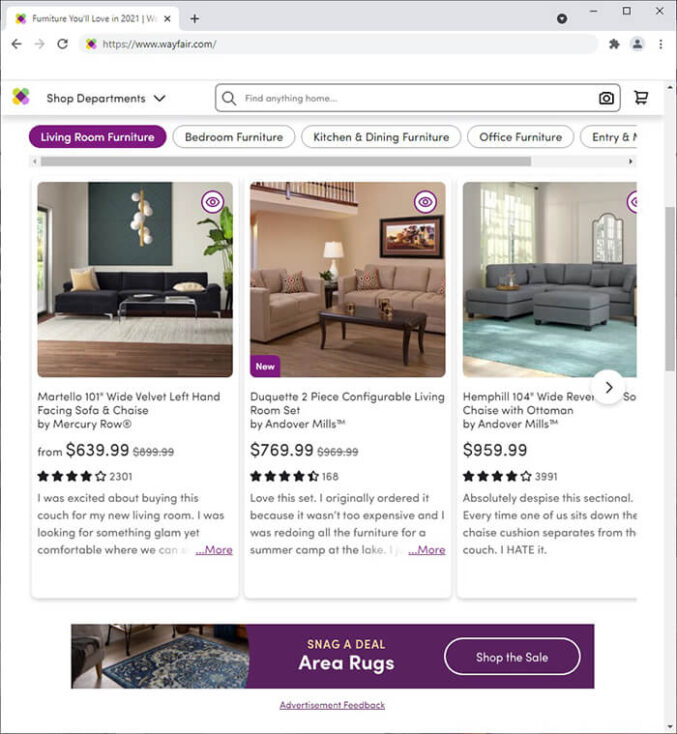Screenshot of a website showcasing various living room furniture options. The browser tab reads, "Furniture You'll Love in 2021 - Wayfair," and the website is www.wayfair.com. The section highlighted in purple is "Living Room Furniture," displaying three featured couches.

1. **Mortello 101-Inch Wide Velvet Left-Hand Facing Sofa by Mercury Row**
   - **Price:** From $639.99
   - **Rating:** 4 out of 5 stars (203.01 reviews)
   - **Description:** A luxurious black velvet sofa perfect for adding a touch of glamour to your living room. Highlights include a left-hand facing design ideal for modern decor. One reviewer notes they were thrilled to purchase this glam and comfortable couch for their new living room.
   - **More Info:** Clickable link for additional details and reviews, indicated by "more" in purple text.

2. **Decor 2-Piece Configurable Living Room Set by Andover Mills**
   - **Price:** $769.99
   - **Rating:** 4.5 out of 5 stars (168 reviews)
   - **Description:** A beige and brown sofa set accompanied by a matching table, white lamp, and a wall painting. This set offers a classic aesthetic suitable for various living spaces. One reviewer shares their satisfaction, noting that the set was affordable and perfect for redecorating their summer camp at the lake.

3. **Healthill 104-Inch Wide Reversible Sofa with Ottoman by Andover Mills**
   - **Price:** $959.99
   - **Rating:** 4 out of 5 stars (391 reviews)
   - **Description:** A grey sofa set featuring a reversible design and an ottoman, ideal for a versatile living space. However, a reviewer expresses frustration with the sectional, mentioning that the cushions frequently separate from the couch, negatively affecting their comfort and experience.